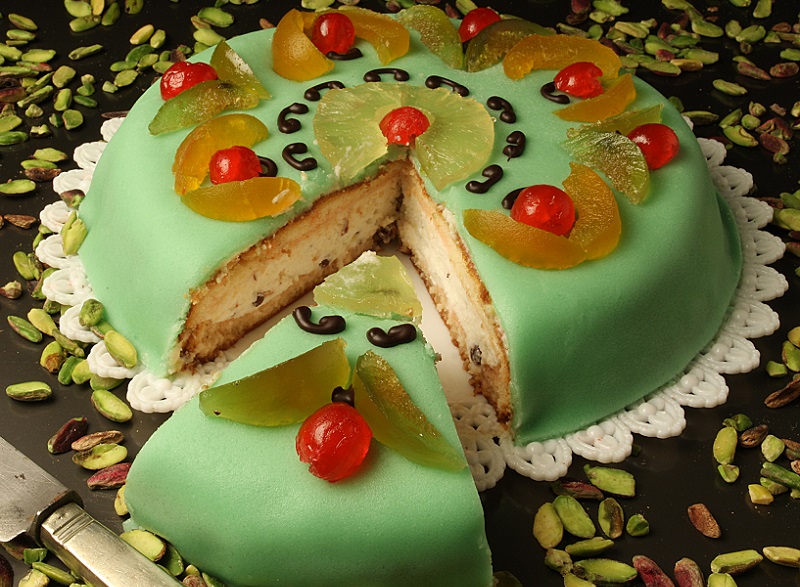The image showcases a visually appealing cake adorned with bright green icing, likely pistachio marzipan, which coats the exterior. The cake's interior consists of layers of creamy vanilla frosting and vanilla cake, though a hint of pink adds an intriguing visual detail. A variety of vibrant fruit slices, including pineapple rings, tangerines, and possibly supremes of oranges, peaches, or apricots, decorate the top alongside bright red cherries positioned both around the center and within a pineapple ring. Scattered around the ornate lacy white plastic plate and the cake itself are numerous pistachio nuts, enhancing the overall aesthetic and complementing the green color. A large slice has been cut and slightly pulled out, revealing the cake’s inner creamy layers. Additionally, small dark chocolate designs and a knife in the corner add finishing touches to this delectable and intricate creation.